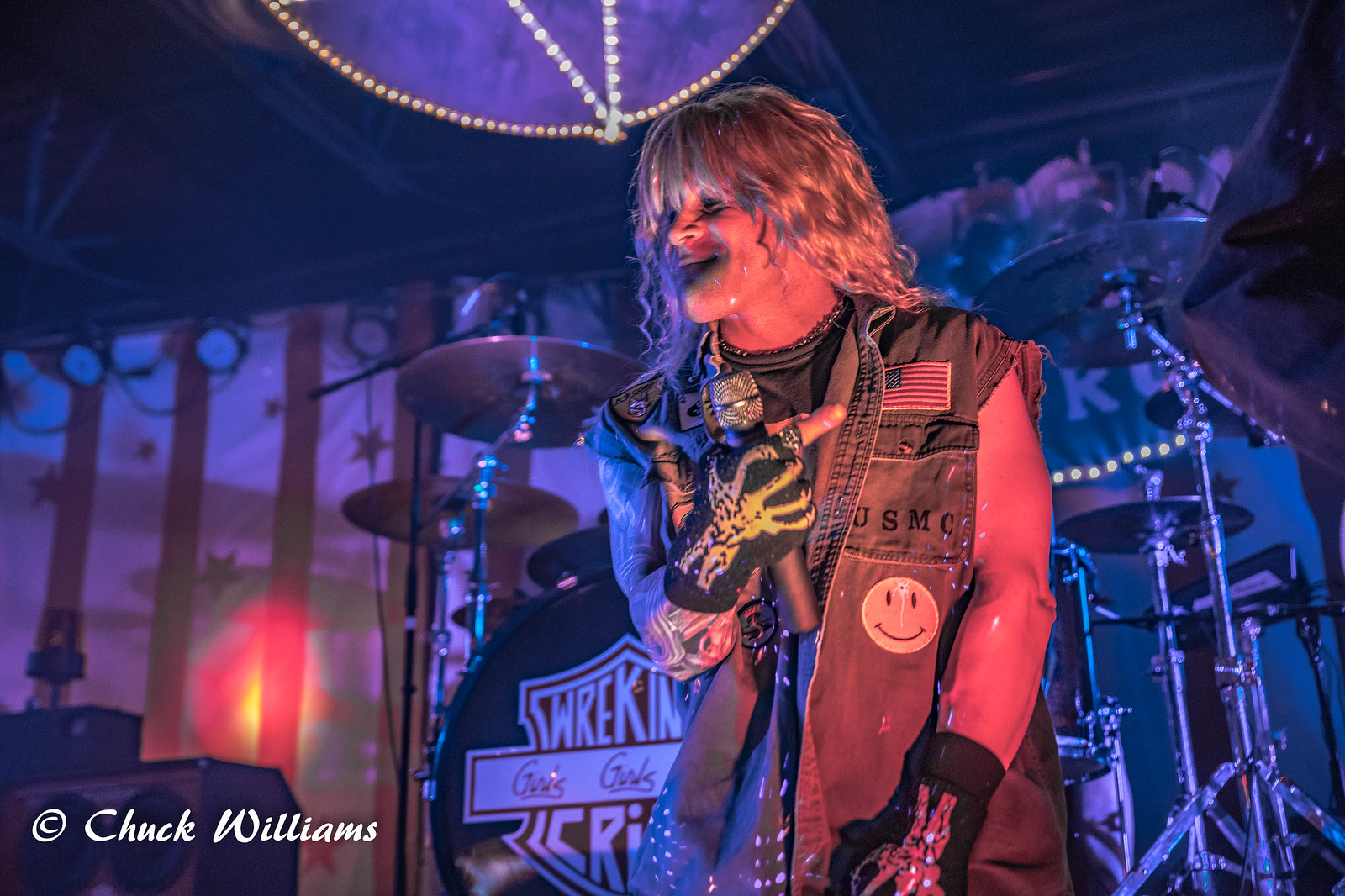The image is a detailed color photograph in landscape orientation capturing a young musician mid-performance on a dimly lit stage, predominantly shrouded in darkness. The performer has long blonde hair that cascades to his shoulders, and he sports striking facial makeup resembling a skeleton mouth. He is adorned in a sleeveless denim blue jacket, conspicuously torn at the sleeves, revealing frayed edges. The jacket is decorated with various patches including a yellow smiley face, an American flag, and stenciled letters reading "USMC." Underneath, he wears a gray shirt. 

On both hands, he dons black gloves with vibrant skeleton hand designs painted on top—noticeably in bright hues of yellow and pink. Clutching a black microphone with a silver top in his right hand, he commands the center stage. The backdrop features a purple and black gothic aesthetic with a round purple light fixture overhead. Visible behind him is a drum set, partially obscured but revealing the letters "W-R-E-K-I-N" alongside partial words like "girls, girls" and "C-R."

In the bottom left corner of the photograph, a watermark reads "copyright Chuck Williams," asserting ownership. The scene is enveloped in a photographic representational realism style, capturing the intense and dramatic essence of the live music experience.